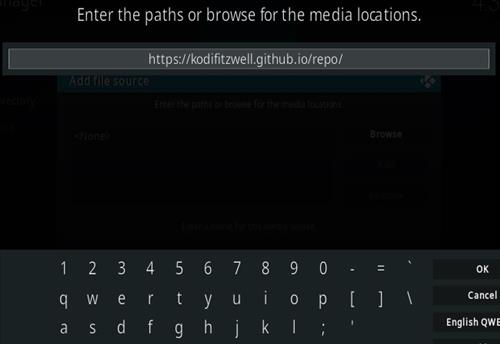This screenshot features a predominantly black background with a few gray elements. At the very top is a light gray, rectangular bar. Directly above this bar, in white text, are the words: "Enter the path or browse for the media locations."

Below this phrase is a darker gray rectangular box with a slight outline. Inside this box, there appears to be a web address that reads: "https://codyfitzwell.github.io/repo/."

Below this box is an empty black space, followed by a numeric and alphabetic keyboard display. The first row of keys includes "1 2 3 4 5 6 7 8 9 0 - =". The second row consists of "Q W E R T Y U I O P [ ] \". The third row contains "A S D F G H J K L ; ' \". Finally, at the bottom right of the image, there are buttons for "OK," "Cancel," and "English (US) QWERTY".